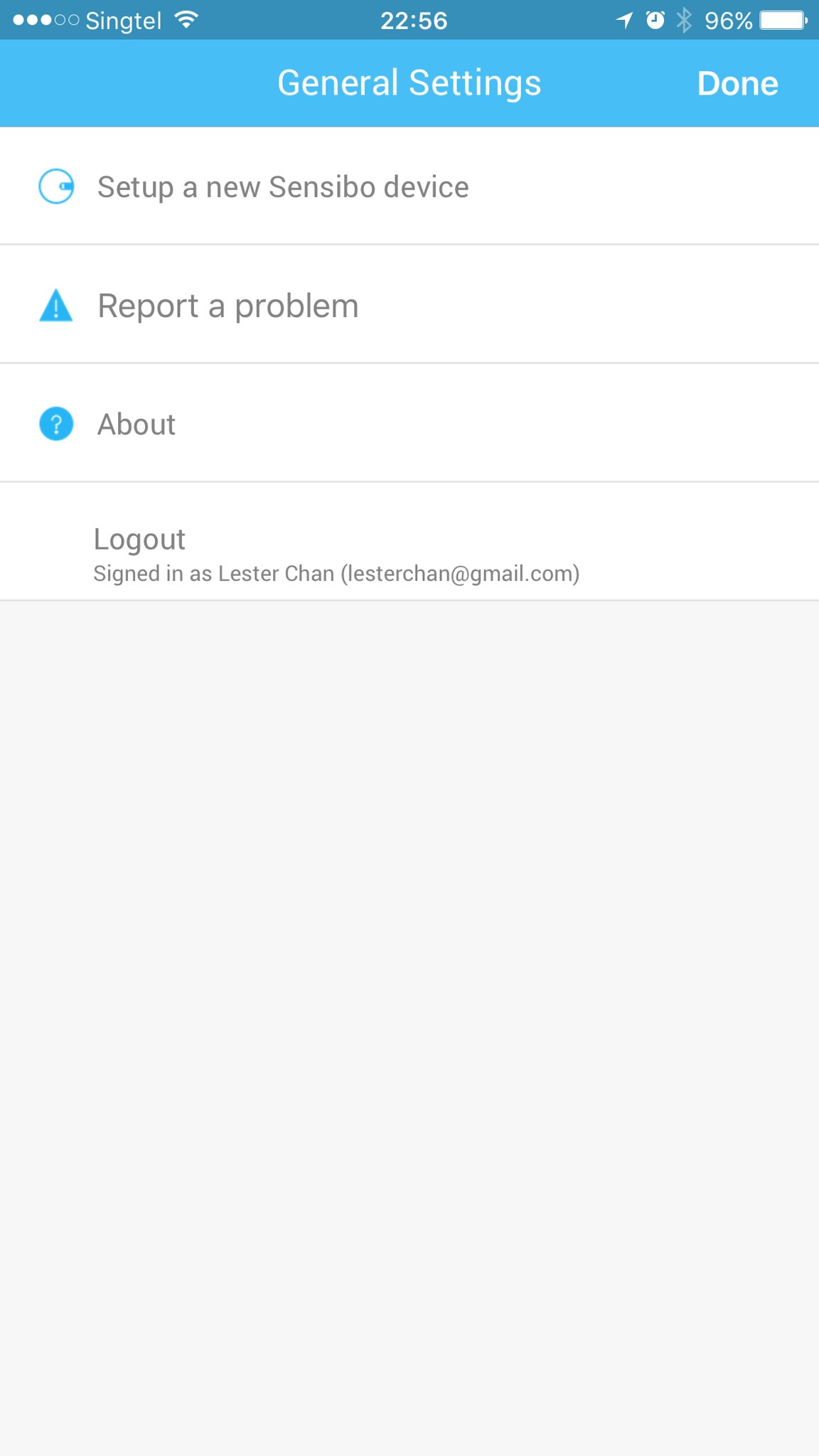The image depicts a smartphone screenshot with a structured user interface. The bottom segment of the screen is a subtle gradient of light gray that almost blends with the white background, providing a minimalistic contrast. 

At the top, a narrow band in medium blue features key status indicators: five dots (three solid white and two outlined) likely representing signal strength. To the right, the label "Singtel" appears, denoting Singapore Telecommunications. A Wi-Fi symbol follows, and centrally displayed is the time "22:56". Continuing rightward, there is a directional arrow, a digital clock icon, a Bluetooth symbol, a battery icon showing 96% charge accompanied by its percentage figure.

Directly beneath this bar, a wider sky-blue banner stretches across the screen with white text, stating "General Settings" on the left and "Done" on the right. The main body of the screen transitions to a clean white background. 

Here, a circular icon labeled "Set up a new Sensibo device" (with the 'S' capitalized) commands attention near the top. This section is demarcated by a thin line below it. Following this, a blue triangle with an embedded white exclamation mark appears next to the text "Report a problem" and is separated by another fine line. Further down, a blue circle containing a question mark is coupled with the word "About". Another thin line precedes the final item, which reads "Logout, signed in as LesterChan (lesterchan@gmail.com)".

This detailed breakdown delivers a comprehensive view of the smartphone's interface at the captured moment.